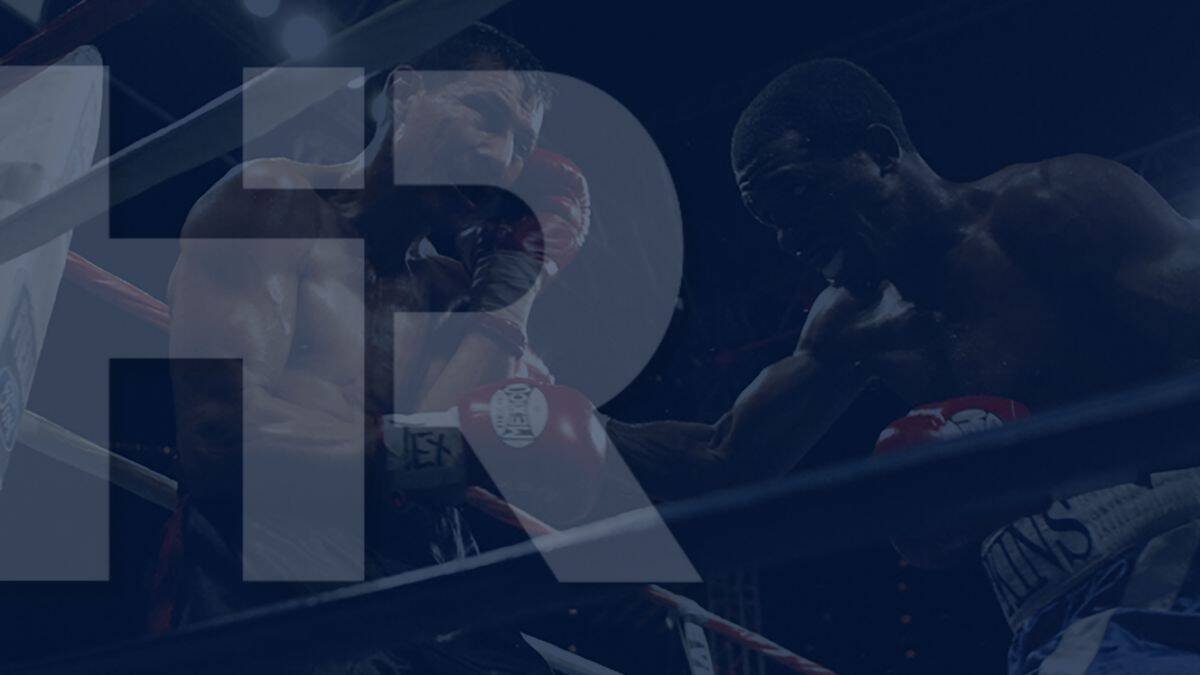The image depicts a dramatic boxing match set against a black background. Two fighters are engaged in a fierce battle within the ring, both sporting red boxing gloves, trunks, and bare chests. The fighter on the left, who appears to be of African-American descent, has longer hair and is pressed against the red and white ropes, his glove raised in a futile attempt to block an incoming punch. The fighter on the right, potentially Hispanic, has very short hair and is in the midst of delivering a powerful blow with his right hand. The impact of the punch is evident, as the fighter on the left wears an expression of pain, with possible cuts on his face, indicating he is on the losing end of the confrontation. Overlaying this intense scene is a white "HR" logo, with the letters intertwined, standing for Hudson Reporter. The image, somewhat shrouded in shadow, underscores the brutal nature of the fight, reminiscent of article discussions on ultimate fighting competitions and their associated injuries.